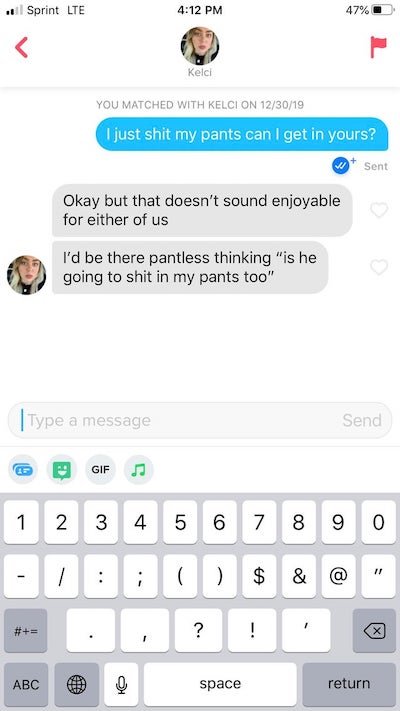A screenshot of a mobile phone screen is displayed with a white background and black text. The mobile carrier at the top left shows "Sprint LTE," and the signal strength icon is next to it. In the center, the time reads "4:12 PM." At the far right top corner, there is a battery icon showing 47% remaining. Below the top bar, there's a horizontal grey line and light grey text stating, "You watched with Kelsey on 12.30.19."

In the main section of the screenshot, there is a detailed image of a woman's head. She has medium skin and blondish hair at the bottom, along with heavy makeup. The accompanying text reveals her name as Kelsey. 

A blue text bubble with white text humorously states, "I just shit my pants. Can I get in yours?" This is followed by blue text indicating that the message was sent. Kelsey’s reply is in a grey bubble: "Okay, but that doesn't sound enjoyable for either of us." Underneath, she further jokes, "I'd be there pantless thinking, 'Is he going to shit in my pants too?'" The back and forth exchange is witty and playful.

Below the conversation are two small heart icons that are grey (indicating they haven't been selected). There is a blank space beneath these hearts, followed by a text input box with a blue cursor. Several grey icons are present within the input field: possibly a GIF symbol, an emoji symbol represented by a green face, and a green music note symbol. The keyboard featured has white keys on a grey background, with darker grey keys at the bottom.